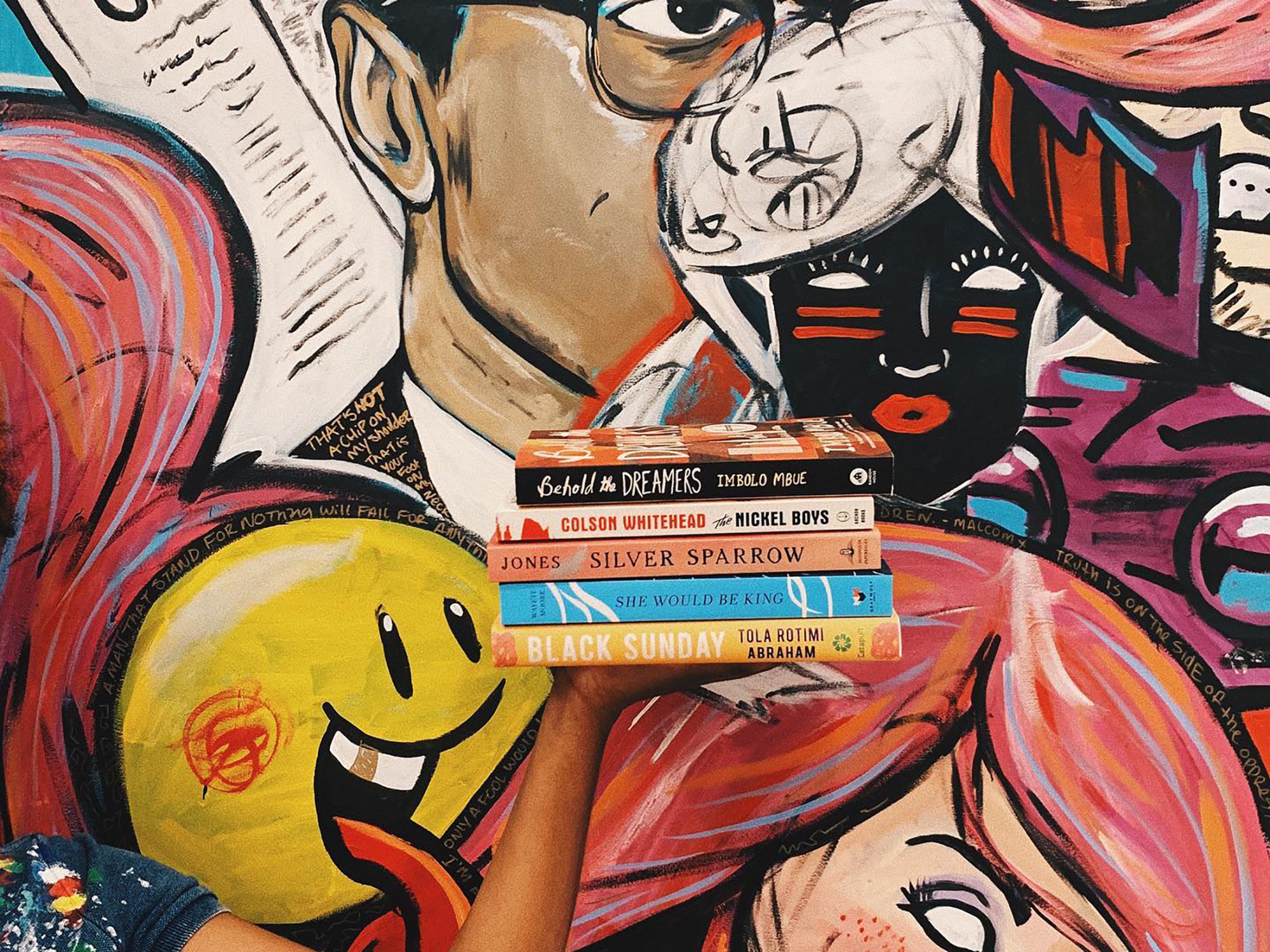In this visually striking photograph, a dark-skinned woman's left hand, clad in a paint-splattered short-sleeved dark blue t-shirt, holds five books aloft in front of an eclectic graffiti-covered wall. The books, from top to bottom, are "Behold the Dreamers" by Mbolo Mbue, "The Nickel Boys" by Colson Whitehead, "Silver Sparrow" by Tayari Jones, "She Would Be King" by Wayétu Moore, and "Black Sunday" by Tola Rotimi Abraham. The mural behind her is an explosion of vivid colors—purple, orange, brown, black, white, and blue accents—featuring a plethora of overlapping images. Among these are a yellow happy face emoji with a tongue sticking out, a portrait of a woman with stark white eyes and flowing red hair, an African-inspired visage with tribal red marks beneath its eyes and red lips, and the partial face of a bespectacled man. Additional elements include a newspaper-like drawing and phrases such as “A man that stands for nothing will fall for anything” and “That’s not a chip on my shoulder, that’s your foot on my neck.” This intricate blend of abstract and realistic art, combined with the human element in the foreground, creates a powerful narrative through its contrasting themes and dynamic compositions.